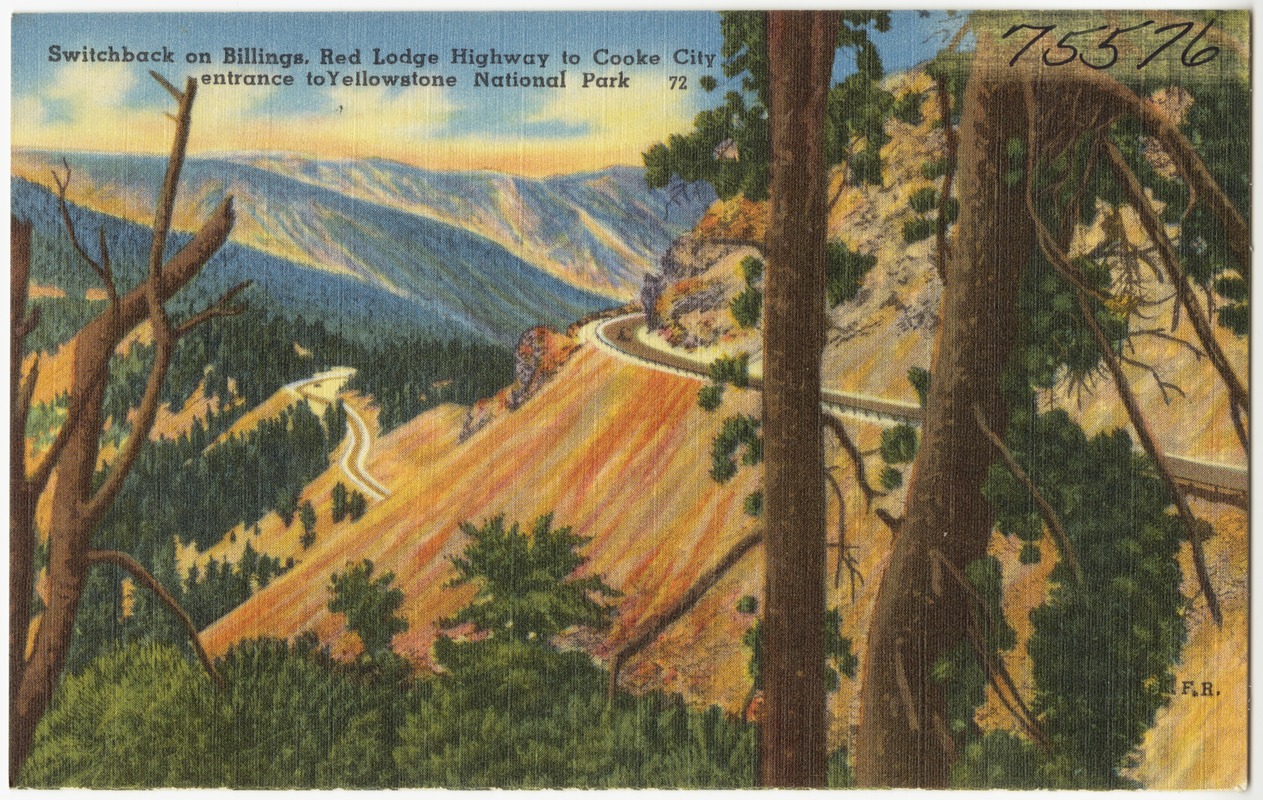This vintage postcard features a colored pencil landscape drawing of Yellowstone National Park, labeled "Switch back on Billings Red Lodge Highway to Cook City, entrance to Yellowstone National Park 72." In the upper right-hand corner, handwritten numbers "75576" are visible. The composition showcases a bluish-gray mountain range to the left and a dark yellowish mountain with a brown roadway carved into it on the right. The foreground is framed by two brown trees, and the image is lined with trees that encircle the scene from the middle left around to the front. Orange soil is depicted below the road, and in the background, snow-covered mountains can be seen further down the canyon. The detailed artistry vividly captures the natural beauty and rugged landscape of this iconic park.